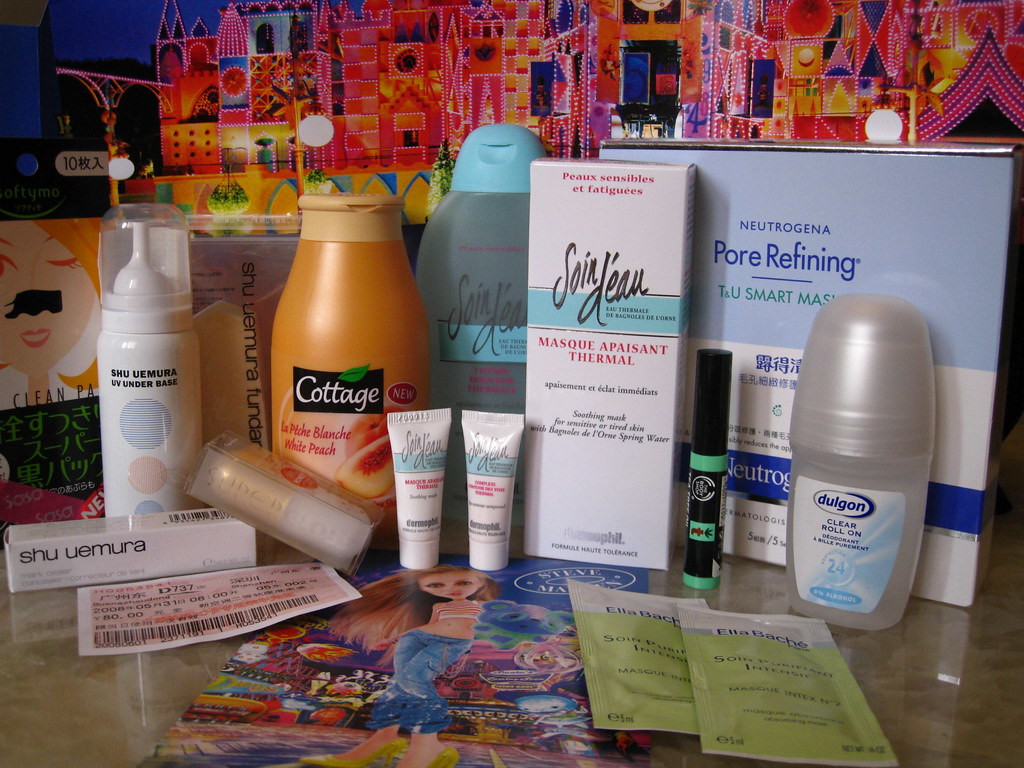This vibrant photograph captures an indoor display of assorted beauty products. The wide, saturated image features a colorful backdrop dominated by shades of orange and yellow, seamlessly blended with hues of blue and purple that evoke an Eastern cityscape reminiscent of "One Thousand and One Nights." Intricately decorated with what appears to be Chinese or Japanese lettering, this backdrop adds an exotic touch to the scene.

The display table in the foreground is laden with a variety of Western beauty products, prominently featuring brands such as Shu Uemura, UV Underbase, Cottage Peach, Swan Dough Mask, and Apeze Tamal. Among them stands a box of Neutrogena Pore Refining products, also adorned with Asian script. Positioned upright along the midline of the photograph are approximately ten of these products, creating a balanced and organized appearance.

Lying flat on the marble counter are additional items, including a flyer depicting a distorted cartoon of a Western-looking woman, which likely serves as an advertisement or promotional material. Scattered packets, possibly face masks, accompany a ticket complete with a barcode and various numbers, adding a layer of intrigue and detail to the scene.

This meticulously arranged display not only highlights the diversity of beauty products but also merges Eastern and Western influences in a visually captivating manner.